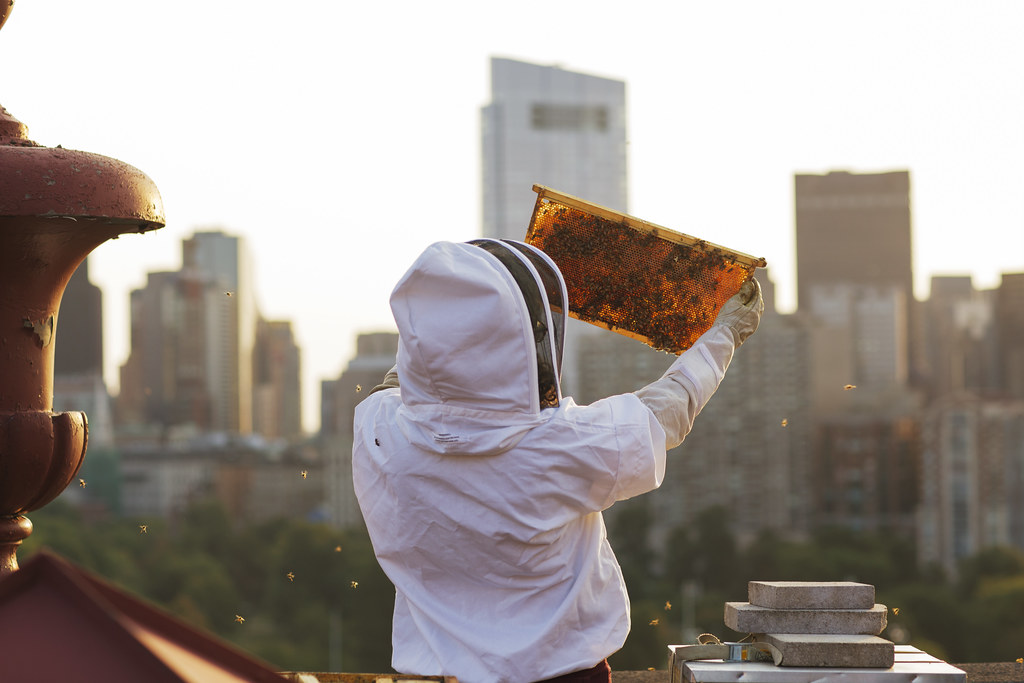In this detailed photograph, a beekeeper, whose gender is indeterminate due to their full beekeeping attire, stands with their back turned to the camera. They are donned in a traditional beekeeping suit which is predominantly white, featuring a cotton hood and a protective black netting that obscures their face. With hands outstretched, the beekeeper holds a rectangular frame teeming with dark brown honeybees, who diligently work on their comb. The comb itself is a rich orange hue, indicative of fresh honey, and numerous bees can be seen buzzing around it. The background reveals a slightly blurry cityscape filled with skyscrapers and buildings, providing a modern, urban contrast to the pastoral activity in the foreground. On the bottom right, three stacked cement slabs are visible, and to the left, there's a faint, cropped-out glimpse of a dark red statue. The overall scene captures a harmonious blend of nature's industriousness within a bustling city.